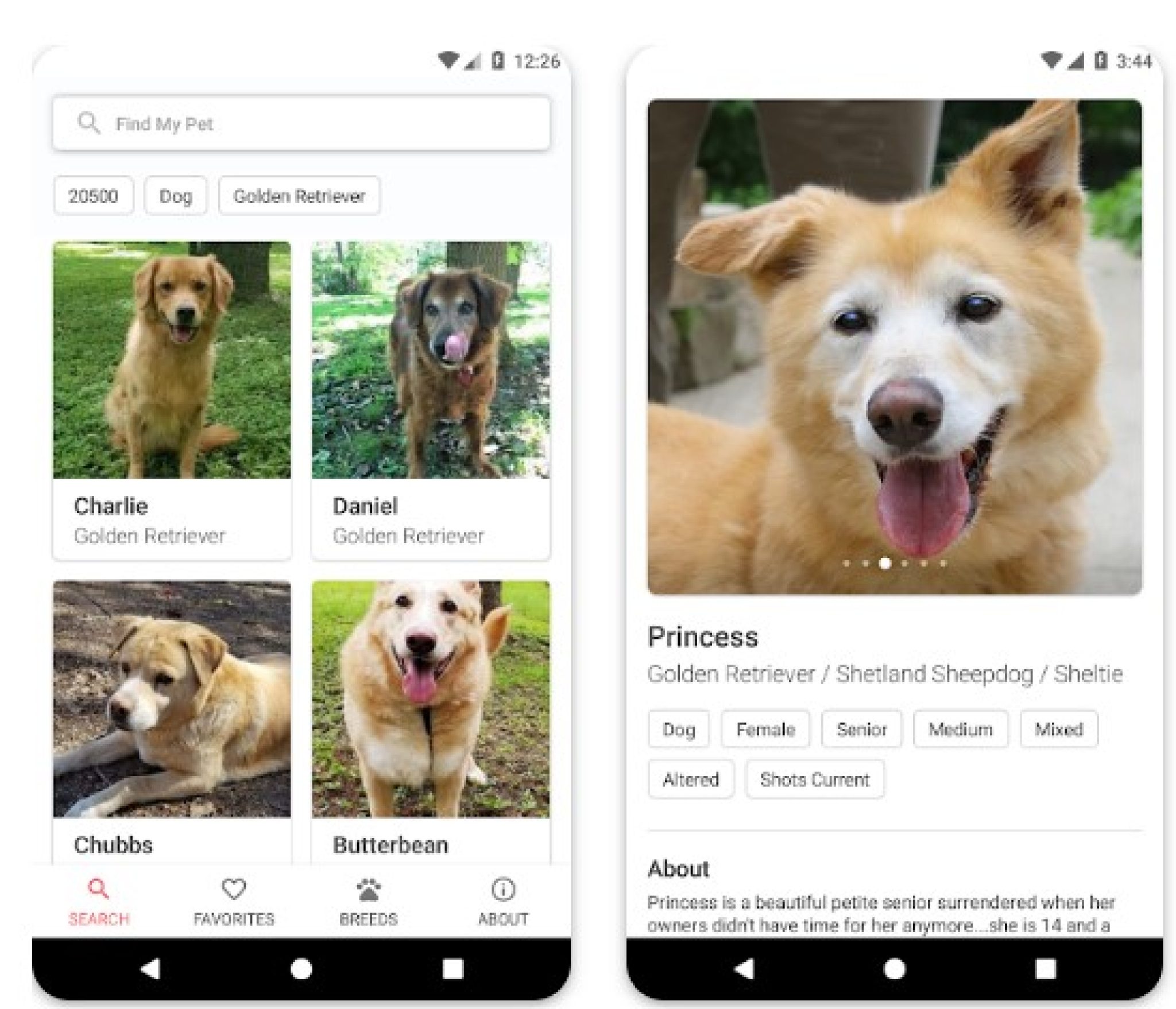The image displays two adjacent cell phone screens featuring a pet adoption app. Both screens show standard status icons including Wi-Fi, cellular signal, and battery indicators, with the times displayed as 12:26 on the left and 3:44 on the right.

On the left screen, the app interface includes a search bar with the text "Find my pet" entered. Below the search bar, there are clickable buttons labeled "20500," "Dog," and "Golden Retriever." Four pictures of dogs are shown in a grid format (two images per row), featuring the names and breeds: Charlie (Golden Retriever), Daniel (Golden Retriever), Chubs, and Butter Bean. At the bottom, there are tabs labeled "Search," "Favorites," "Breeds," and "About," along with navigation icons for home (circle) and recent apps (square).

The right screen showcases a detailed profile for a dog named Princess, described as a "Golden Retriever Shetland Sheepdog Sheltie mix, Female, Senior, Medium, Mixed, Altered, Shots current". The bio explains that Princess is a petite senior who was surrendered by her owners due to lack of time for her care. She is 14 years old. The app provides multiple photos of Princess, allowing potential adopters to swipe through her images. The app seems dedicated to pet adoption, offering extensive details about each pet to help users find a suitable companion.

This app functions similarly to a pet finder, not for recovering lost pets, but for locating pets available for adoption. It features a variety of pets with detailed profiles, aiding potential adopters in making informed decisions.